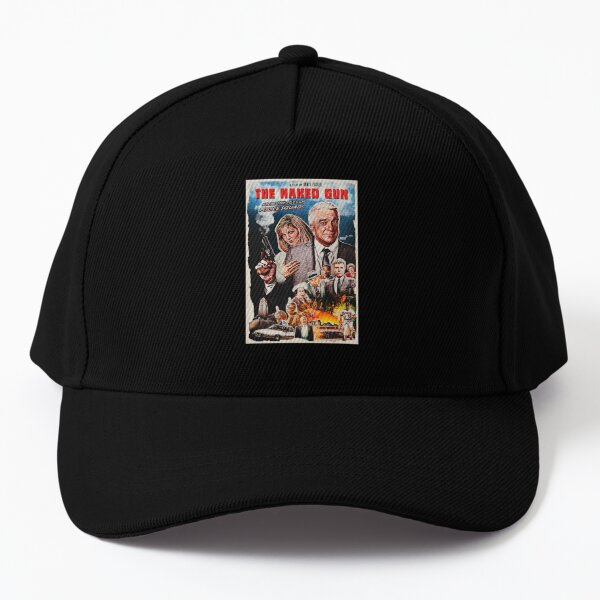This image features a pristine black baseball cap, prominently displayed against a white background that accentuates its dark hue. The cap appears unworn and well-constructed, with visible stitching and a small button on top. The focal point of the cap is the front panel, which showcases a design modeled after "The Naked Gun" movie poster. Dominating the center of this design is the title "The Naked Gun" in bold red font. Beneath the title, a retro-style illustration depicts an older man with white hair in a suit, holding a smoking gun, with his companion, a blonde woman, standing beside him, her hand resting on his shoulder. Smaller figures and additional imagery, including a cluster of characters, cars, and what seems like an explosion or fire, are situated towards the lower portion of the design. This detailed artwork underscores the cap's cinematic theme, making it an eye-catching and unique accessory.